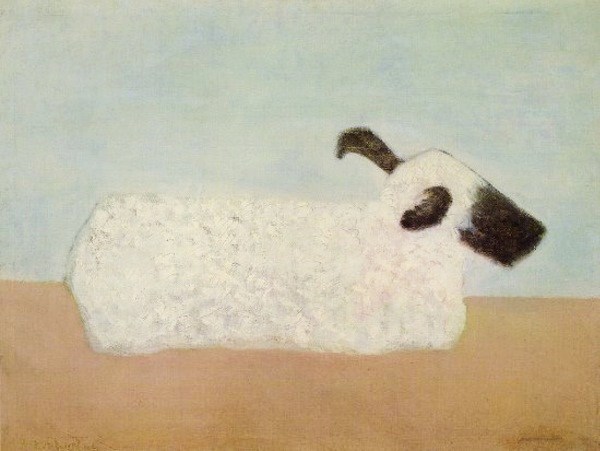This image is a child-like painting characterized by its simple and somewhat abstract style. The top half of the painting features a plain white sky with touches of blue, while the bottom third is dominated by a brown horizontal line, representing the ground. In the center of the brown ground lies a simplified, undefined white form resembling a sheep or possibly a steer, hinting at an animal resting with its legs curled underneath it. The creature has prominent black details including two ears – one ear pointing towards the viewer and the other back towards the white sky – as well as a black snout and mouth. No eyes or fine details are discernible, contributing to the overall vague and blurry appearance. The animal's back seems rounded, and there are no visible legs or tail, further emphasizing the basic artistic style of the painting.